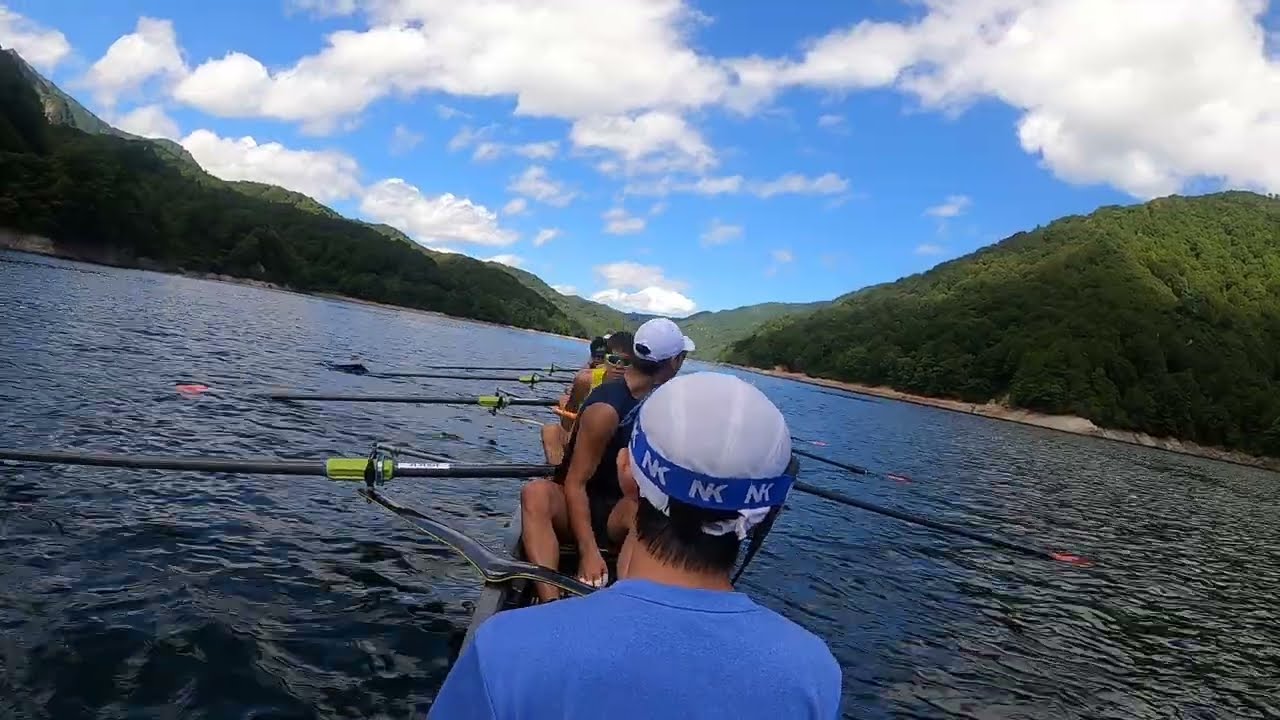In the photograph, a rowing team is seen navigating across a serene mountain lake under a clear blue sky dotted with white, puffy clouds. The team is positioned vertically from the bottom to the top of the image. The individual closest to the camera, wearing a blue t-shirt and a white hat inscribed with "NK," has a strap around his head and is facing forward. The second man, dressed in a black tank top and a white baseball cap, is turned slightly to look back. Further up, a third rower in a yellow tank top and sunglasses faces the camera. The fourth man is partially obscured but visible. The athletes grip their oars, which have gray blades trimmed with yellow or white. Majestic, forested mountains frame the lake on both the left and the right, with a particularly ridged hill on the left and a more rounded one on the right. In the distance, additional hills enhance the picturesque scene.